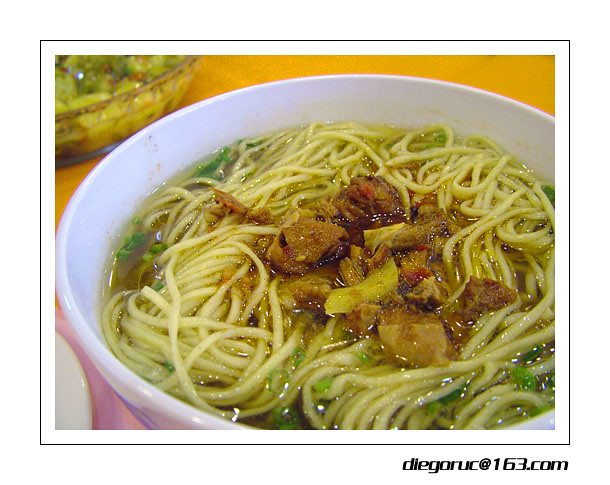The image features a close-up of a bowl of ramen soup, bordered by a thin white and black line, with the text "diegoruc at 163.com" located in the bottom right corner. The soup, set in a white bowl, is filled with tan ramen noodles immersed in a light, clear broth. Green onions are sprinkled throughout, adding a splash of freshness. At the center of the bowl, pieces of brown meat and various vegetables are visible. The photo’s soft, inviting tones are complemented by the light orange and pink tablecloth below. Another blurred dish is partially visible in the top left corner, suggesting the setting is part of a meal. The angle of the photograph gives a downward perspective, capturing the appetizing details of the dish.